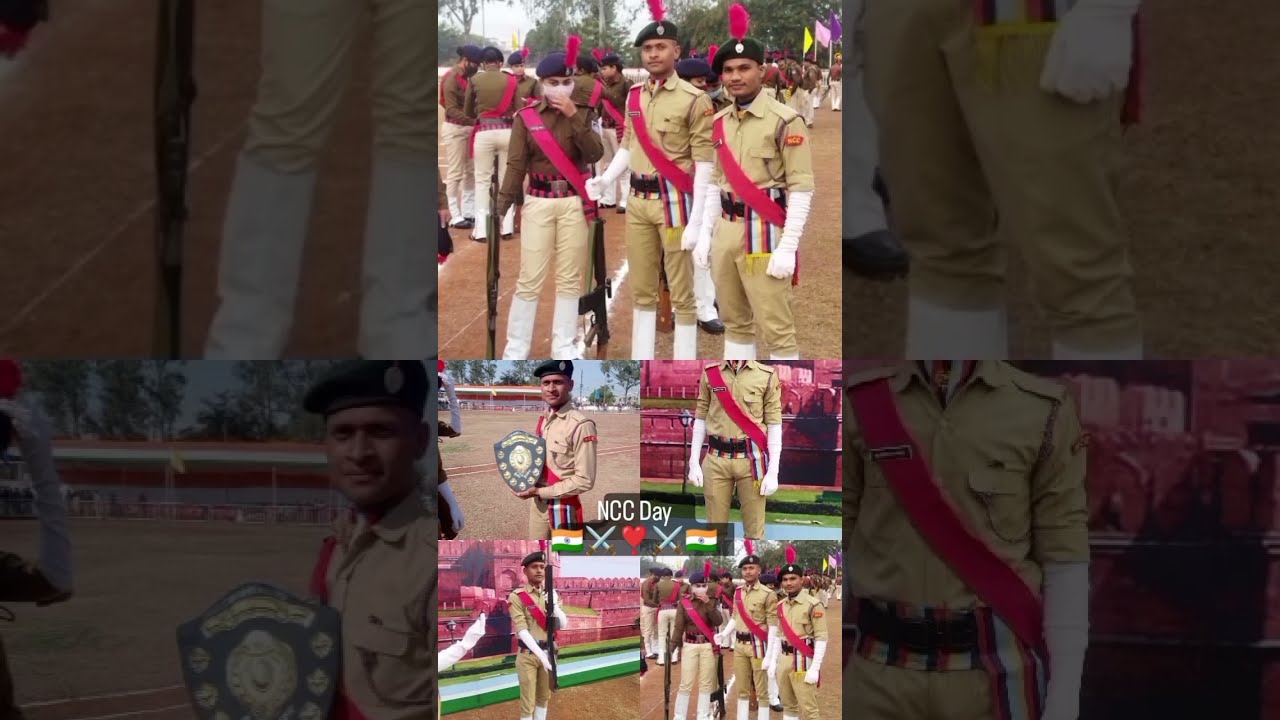The image is a color photograph collage in portrait orientation, centered on an enlarged and darkened version of the same photo, which acts as the background on either side. The main collage is divided into one large top photo and four smaller photos arranged in a 2x2 grid below it. The top photo features three young military officers from a Middle Eastern country dressed in striking parade uniforms. They wear tan outfits adorned with a red sash across the right shoulder, long white opera gloves, white leggings, and white boots. Their uniforms are completed with dark-colored berets featuring red feather plumes. Behind them, other soldiers are engaged in casual conversation amidst a backdrop decorated with colorful flags—purple, blue, lavender, yellow, and red. The grid below includes close-up snapshots: one of a soldier holding a black and gold shield-shaped plaque, another of a soldier standing solo for a portrait, a third of a soldier bearing a flag, and a fourth presumably of another officer. Over the center of the collage reads "NCC Day" in bold lettering, flanked by two Indian flag emojis, a heart, and crossed swords beneath. The detailed and representational style of the photos captures a vivid moment of a ceremonial military event.